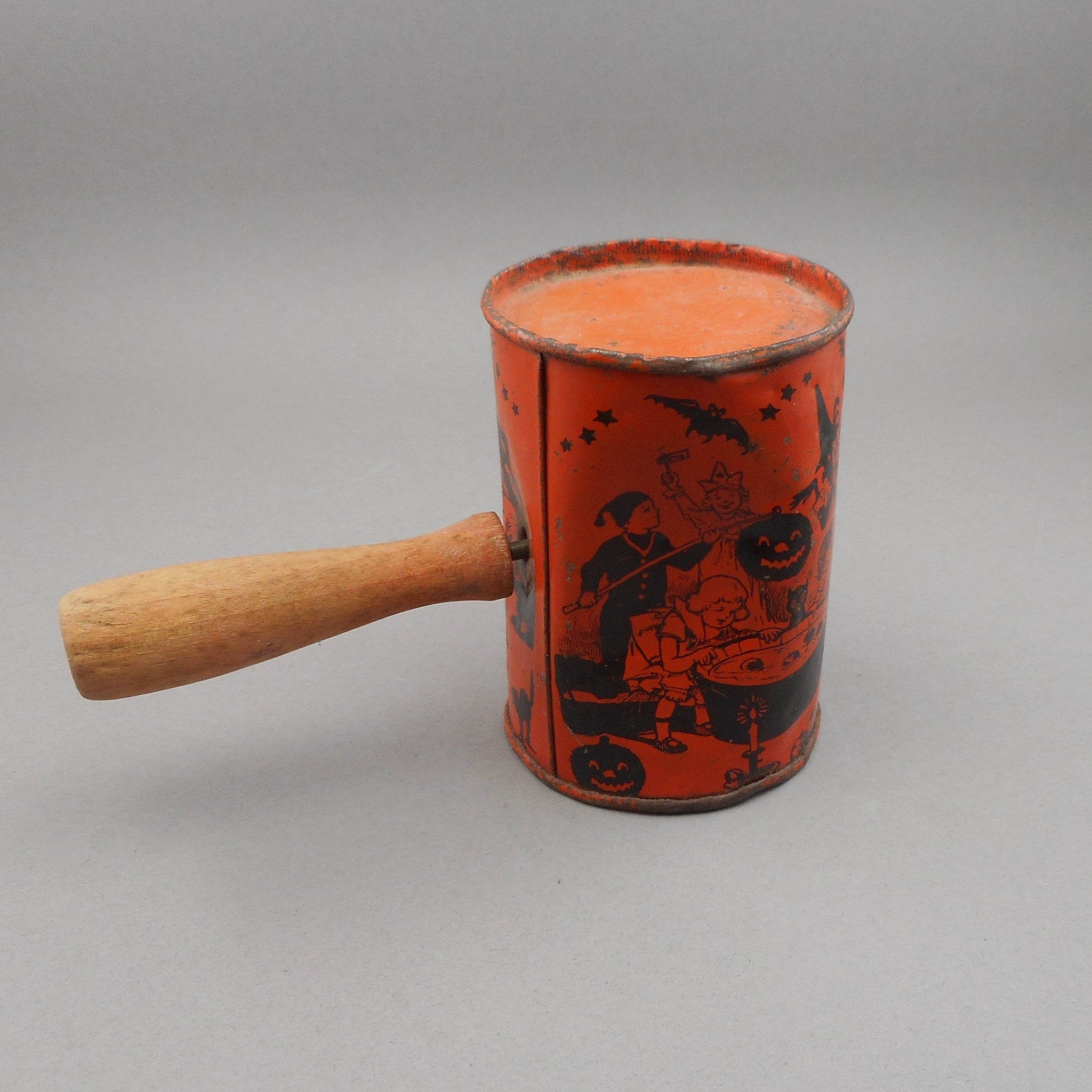The image depicts a distressed, vintage Halloween-themed object resembling a hammer or a gavel. The head of the hammer seems to be a repurposed, old-fashioned orange can adorned with black painted designs. The can is worn, revealing patches of rusty aluminum beneath the orange paint, and it is mounted on a long wooden handle that appears to pass through the side. The painted black designs on the can include a smiling pumpkin, children in old-fashioned clothing (some of whom appear to be bobbing for apples), stars, a flying bat, and additional Halloween motifs. This object is set against a flat, gray background with no visible text.